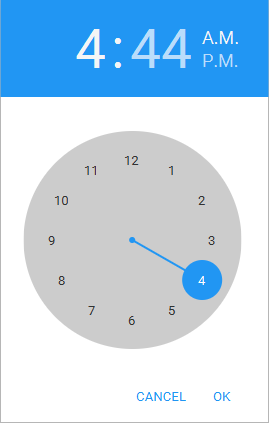A screen capture depicting a digital clock interface likely from a mobile app or a Windows program. The upper section of the image features a blue horizontal rectangle displaying the time as "4:44 AM." The "4" for the hour is in white, while the "44" for the minutes is in light blue. The "AM" indicator is in white and is stacked vertically alongside an identical "PM" indicator, suggesting it's 4:44 a.m.

Below this digital display is a traditional clock face with a single hand pointing to the 4 o'clock position. The hour hand is blue and is highlighted by a blue dot at the 4 o'clock mark, where the number "4" is prominently displayed in white. The rest of the clock face is gray, and the other hour markers are black.

In the lower right corner of the interface are buttons labeled "Cancel" and "OK" in blue capital letters. The lower three-quarters of the image has a white background, and the entire image is outlined with a thin black rectangle. It's clearly showing the time as 4:44 a.m. with only the hour hand visible on the clock face, and no minute or second hands present.